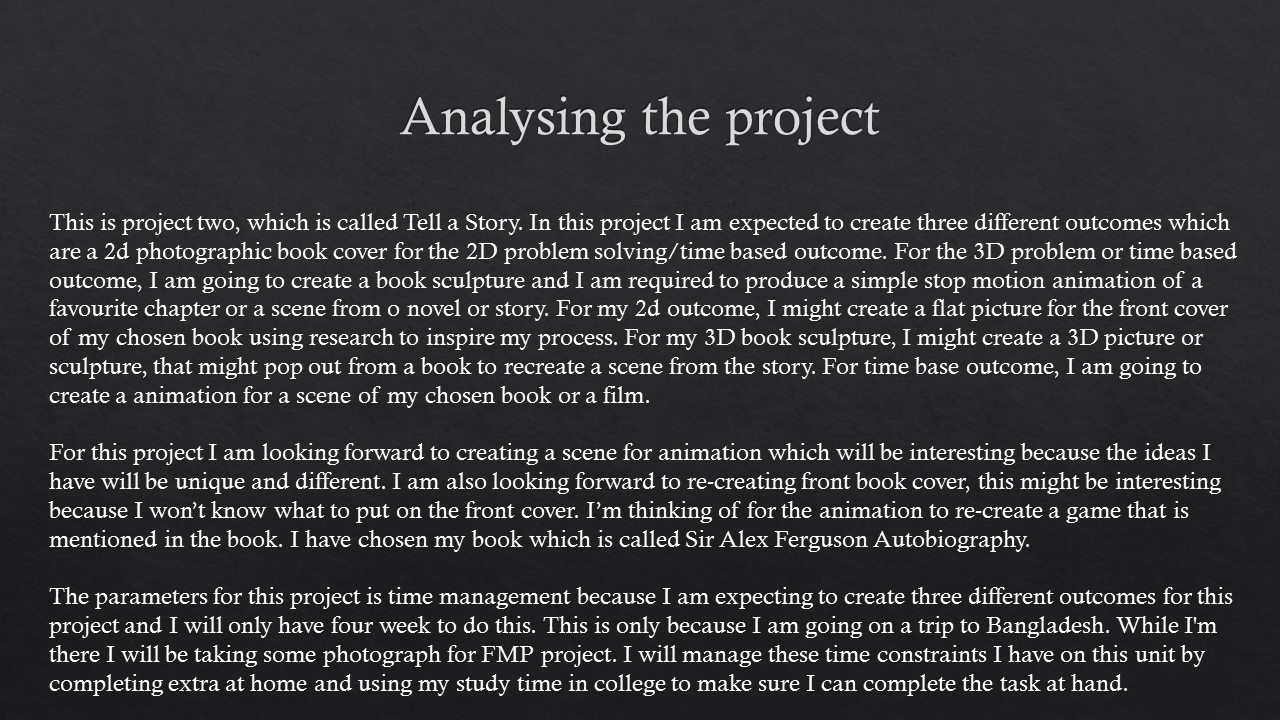The image features a screenshot or possibly a printed document titled "Analyzing the Project," presented in bold white text on a black background. The document outlines Project 2, named "Tell a Story," which involves creating three distinct outcomes. The first paragraph details that the outcomes include a 2D photographic book cover for a 2D problem-solving or time-based task, a book sculpture for a 3D problem-solving task, and a simple stop-motion animation of a favorite chapter or scene from a novel or story. The second paragraph elaborates on the intent to create a flat picture for the book's cover, using research to inform the process, and a 3D picture or sculpture that might pop out from the book. The third paragraph highlights time management as a critical parameter, mentioning a limited four-week timeframe and an impending trip to Bangladesh to take photographs relevant to the project.